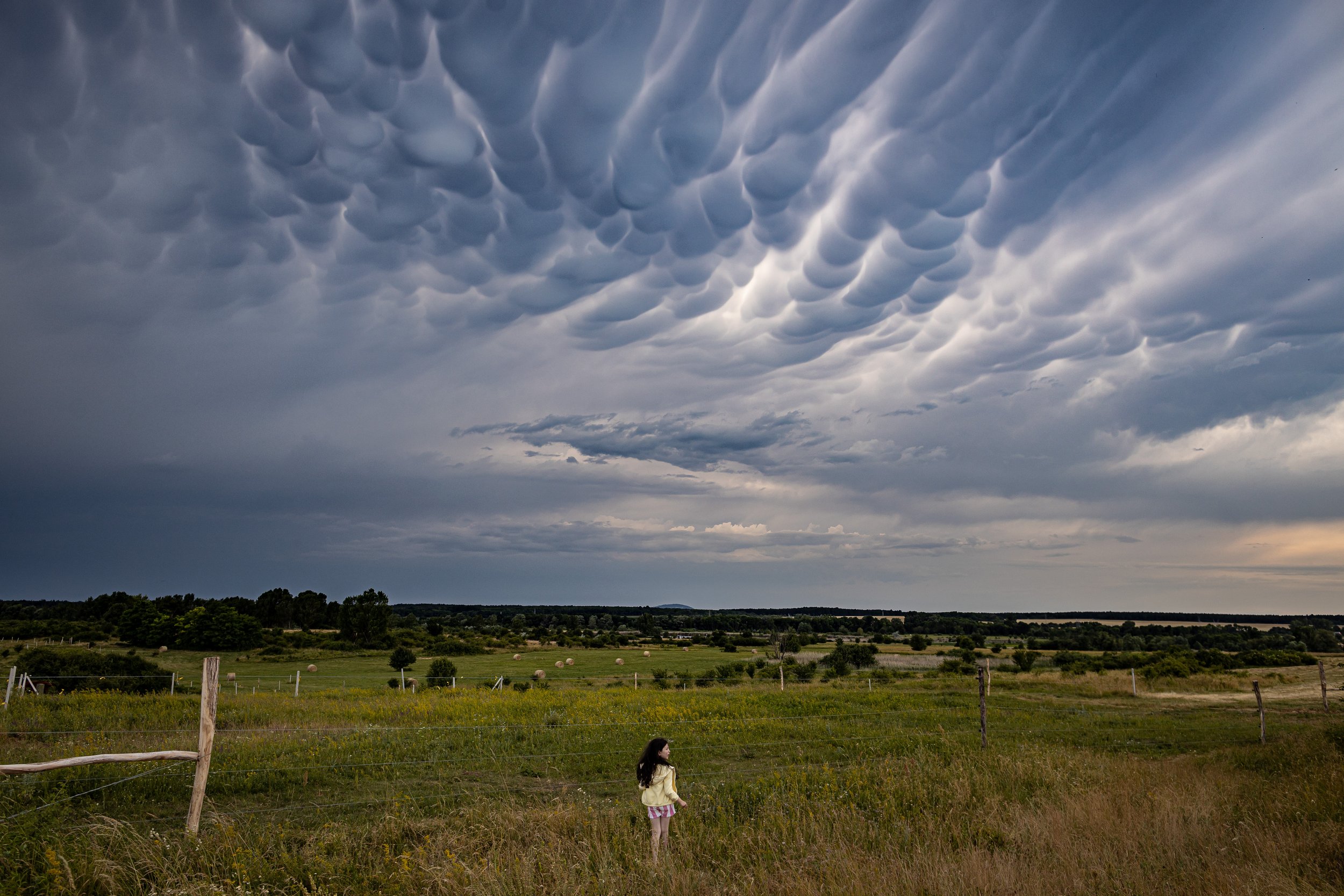The image depicts a striking scene beneath a stormy sky, where mammatus clouds dominate the upper two-thirds of the frame, creating a dramatic and turbulent atmosphere. Sheets of rain can be seen in the lower left, stretching towards the horizon, enhancing the sense of an impending severe storm. Below this tumultuous sky lies a remote farm field, characterized by short to medium-sized grasses and clusters of yellow wildflowers. Scattered wooden posts and sections of barbed wire fencing suggest a rustic agricultural setting, possibly with an electrical fence partially visible. Hay bales are dotted across the field, left to dry after harvest. In the center stands a young woman with long black hair, her light yellow long-sleeve outfit catching what little light pierces the overcast sky. She appears to be wearing a checked skirt, possibly of purple and white, or pink shorts. She is gazing upwards and to the right, seemingly mesmerized by the storm clouds, while her hair is gently tousled by the wind. The scene exudes a lonely yet serene atmosphere, with the woman standing solitary amid the wild, untamed beauty of the landscape.